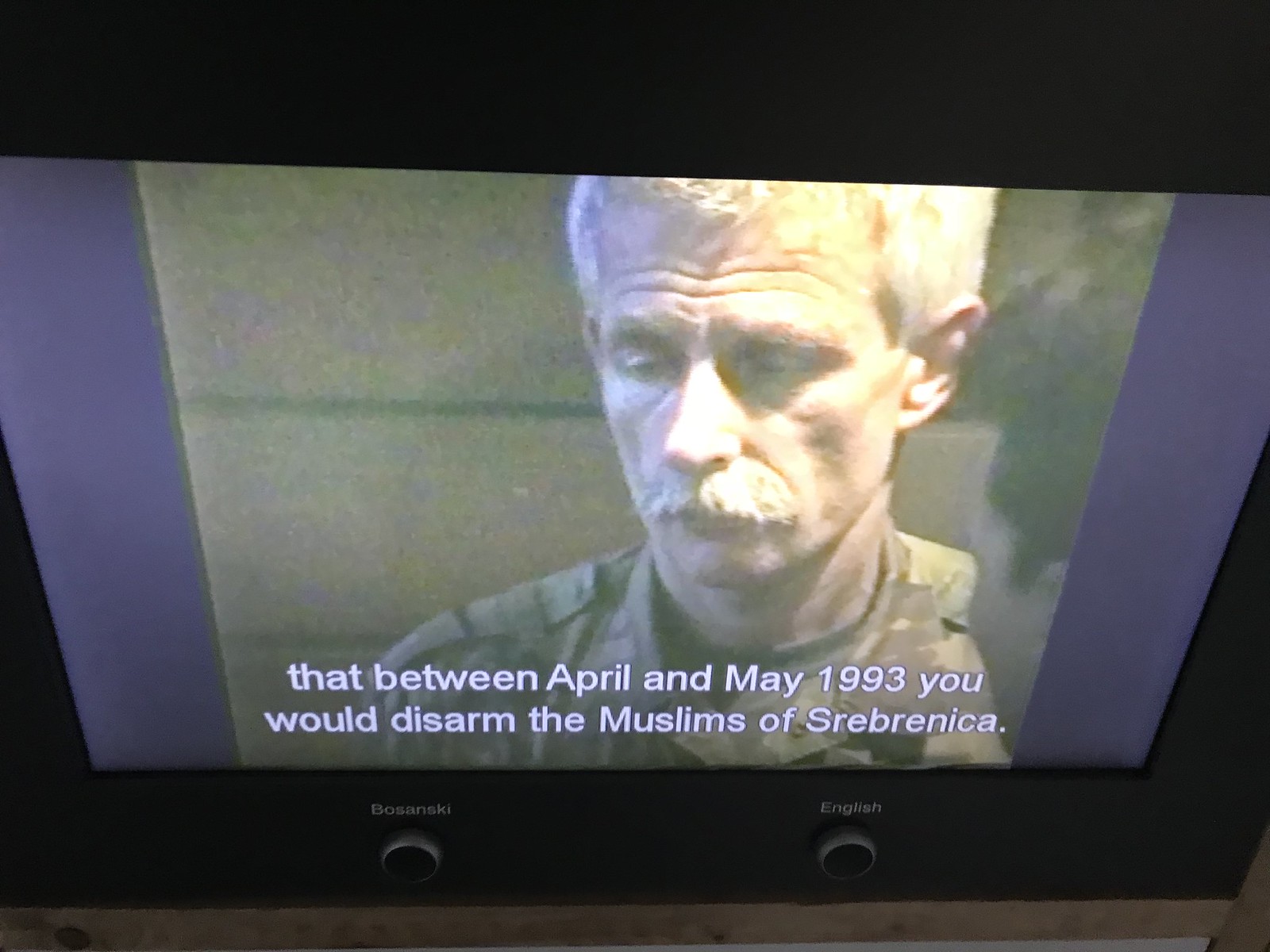This image depicts a small electronic screen, possibly either a digital frame or a low-resolution monitor. The device has a black outline and features two circular buttons at the bottom; the left button is labeled "Bosanski" and the right is labeled "English." The primary content on the screen is a photograph of an older Caucasian man, indicated to be in a military uniform with gray hair and a small mustache. Visible on the right side of the photo is the partial face of another individual. Beneath the photo, a white subtitle states, "Between April and May 1993, you will disarm the Muslims of Srebrenica." The screen does not appear to display its content optimally, as the image quality is low and possibly taken in dim lighting, contributing to the overall unclear presentation.